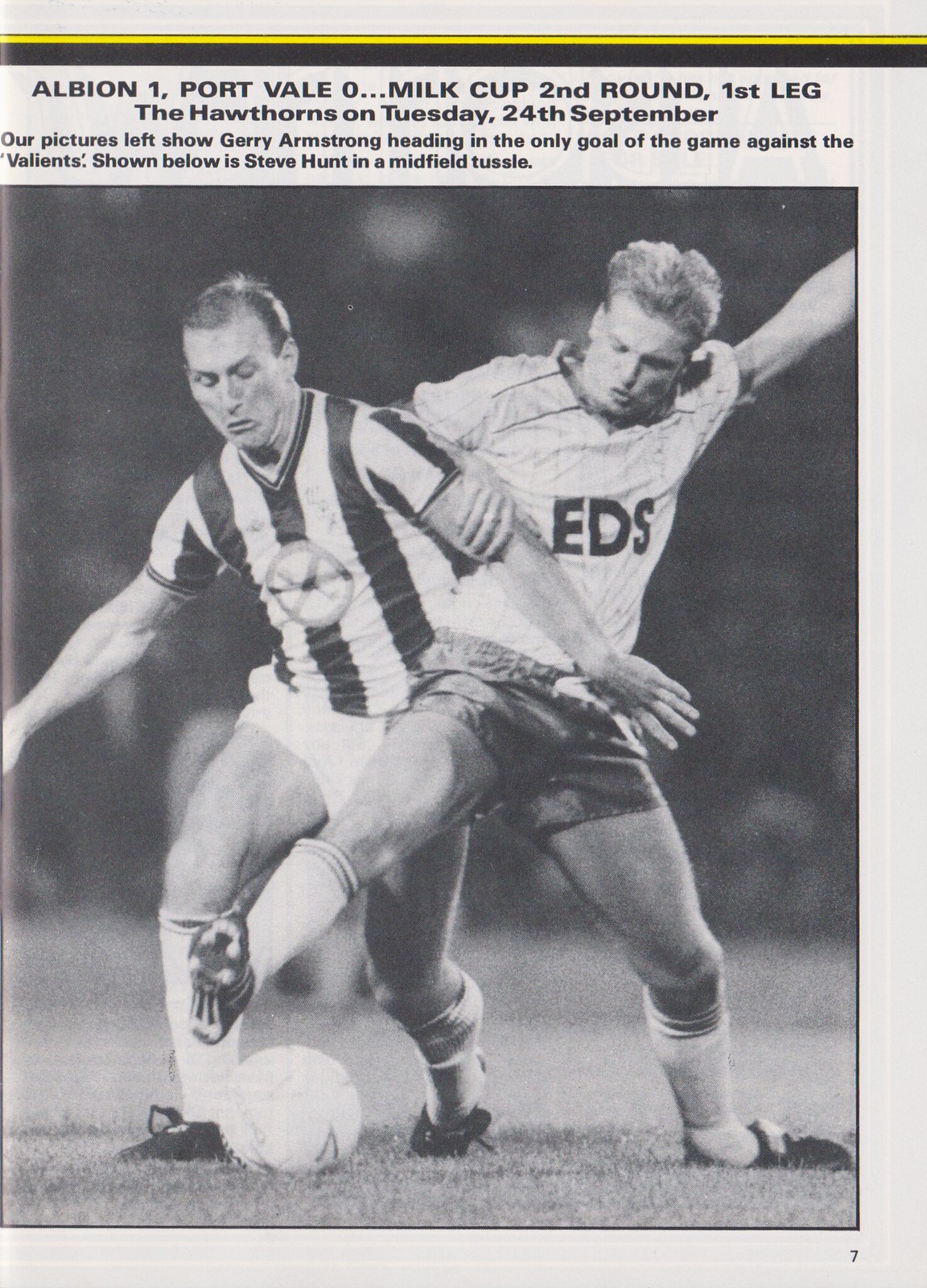This black-and-white newspaper clipping features a central photograph of two soccer players in a dynamic struggle for control of the ball on a grassy field. The player on the left has his left arm positioned in front of his opponent’s torso, while the player on the right extends his right leg over the left player's hip. This intense midfield tussle captures the competitive spirit of the match. Above the image, black text on a light background under a black bar reads: "Albion 1, Port Vale 0, Milk Cup, Second Round, First Leg, The Hawthorns on Tuesday, 24th September." The caption highlights Jerry Armstrong heading in the only goal of the game against the Valiants, and features Steve Hunt engaging in the visible midfield struggle. The overall aesthetic suggests it is a page taken from a sports section of a newspaper, detailing the significant moments of the game with vintage tones of tan, yellow, black, and different shades of gray.